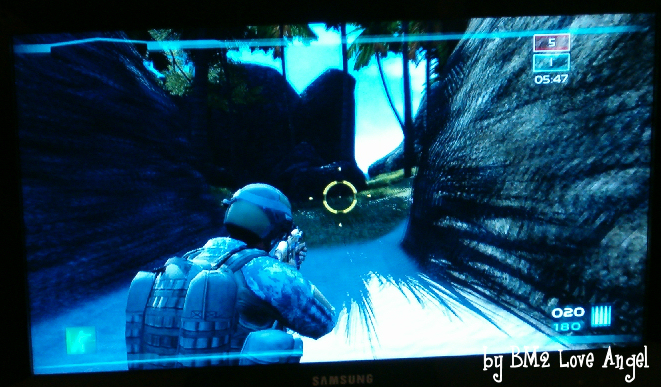This detailed screenshot from a video game, displayed on a Samsung monitor, showcases a soldier clad in a helmet and heavy vest, holding a gun pointed at a yellow circular target with white dots. The soldier, also wearing a blue backpack, stands on a dirt road flanked by large dark rocks. Above him, tall palm and leafy trees rise into a clear blue sky dotted with white clouds. At the top of the screen, a red square with the number '5' and a blue square with the number '1' are displayed, followed by the time '05:47.' At the bottom right, white text reads, "BYE BM2 LOVE ANGEL."